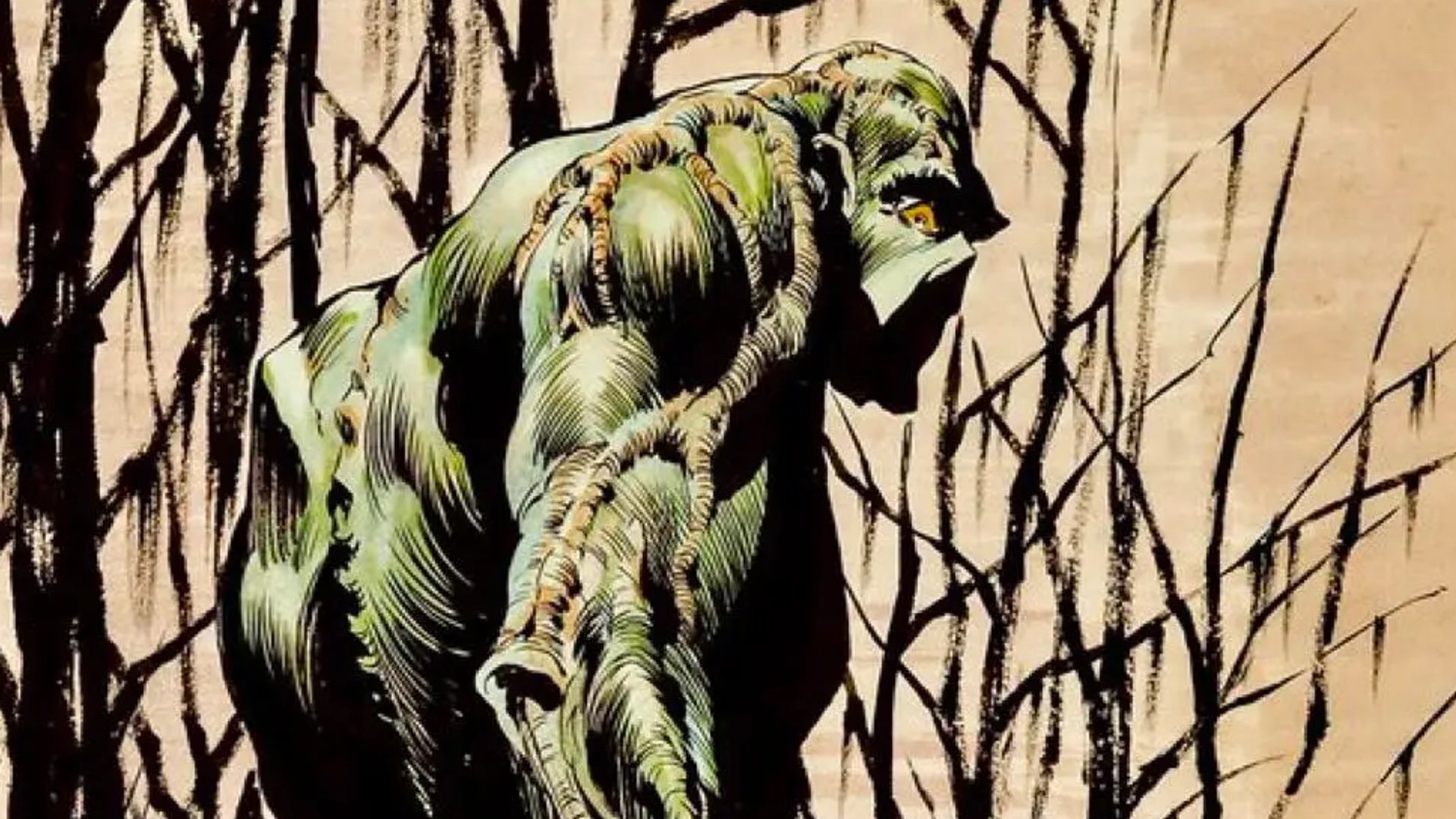The artwork is a detailed and brooding depiction of Swamp Thing, captured through an intricate sketch. The green, imposing creature emerges from the marshes, framed by hanging mossy vines that form a rich, tangled background. His skin is meticulously rendered with pronounced, twisted, and raised webbing along his arms and across his back, resembling tree branches. Adding to this organic texture are brown and black tints that accentuate his muscular, veiny form, almost mimicking the vascularity of an ancient tree. Swamp Thing's yellow, amber-colored eyes peek back at us over his right shoulder, set against a daytime backdrop with hues of yellow, brown, and pinkish tones, populated by wispy trees and branches. The attention to detail, from the furrowed lines in his skin to his looming, haunted gaze, creates a vivid and captivating portrayal of the swamp creature.